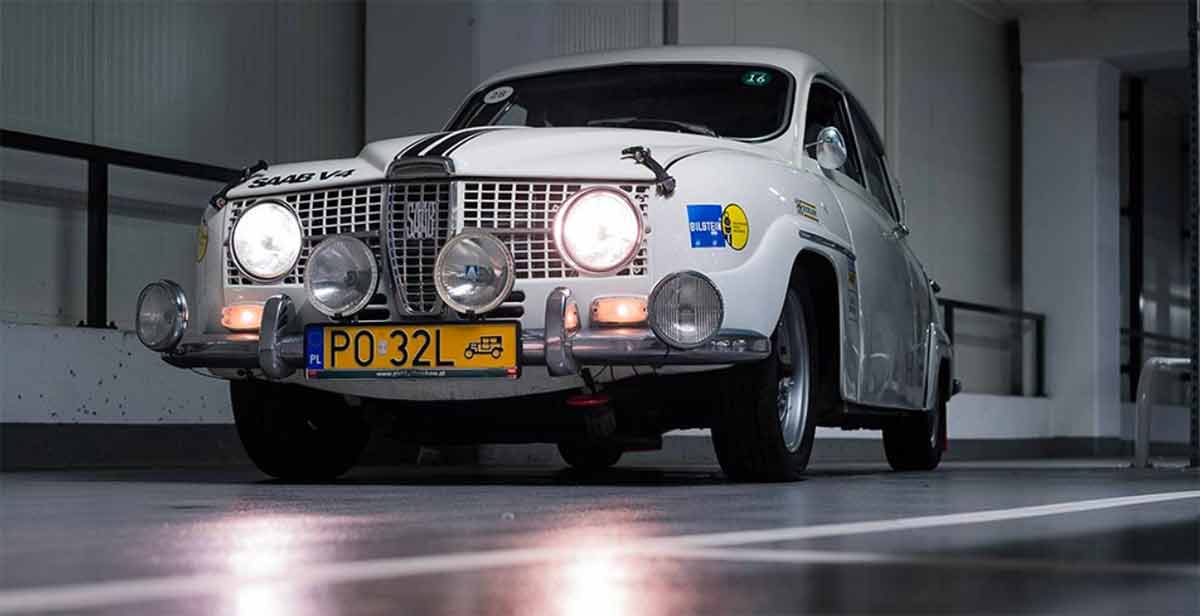This image features a white Saab V4 automobile prominently displayed in what appears to be an industrial showroom setting. The car, which is photographed at a ground-level perspective and facing the viewer, has its headlights illuminated, casting reflections on the ground that suggests a wet or smooth surface, possibly concrete or metal. A notable feature on the hood is black racing stripes, with "Saab V4" inscribed in black lettering near the left headlight. The vehicle is equipped with a silver front grille, black wheels with silver rims, and a distinctive yellow license plate, marked with P032L, indicative of a European style plate.

The background of the image shows a structure with a primarily white wall that stretches about three-quarters across the frame, accompanied by metal siding and glass windows with gray trim. There is a vertical pillar at the corner and another horizontal pillar that extends from it. The environment is characterized by its grey and white industrial aesthetics, complemented by metal guardrails on the adjoining walkways. The picture seems to be taken at nighttime, further accentuating the illuminated headlights and the reflective qualities of the surroundings.